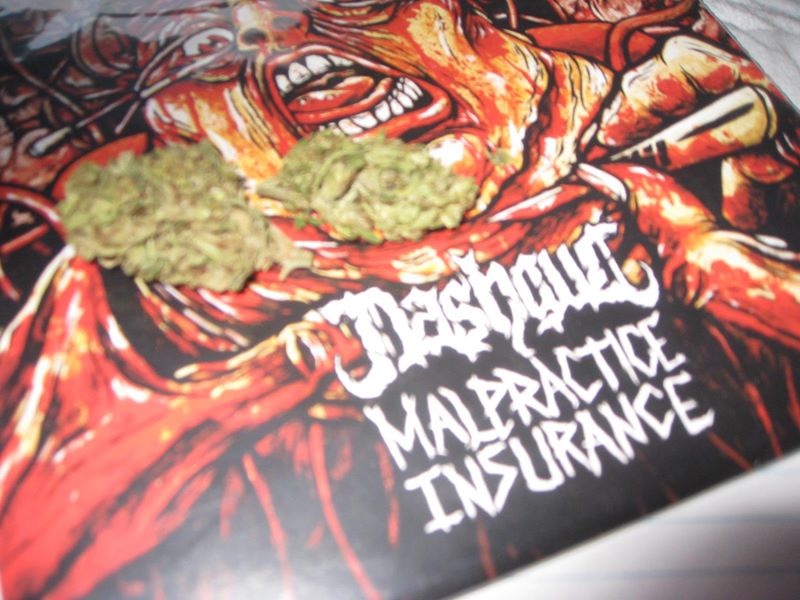This photograph showcases a striking and unsettling piece of artwork depicting a gory cartoon face with red eyes and an open mouth, apparently representing a demon. The face is bloodied, with blood also covering the neck and body, and red hands with long white nails reaching out from the bottom of the image. The artwork is not centered in the frame and is tilted at an angle, partially obscured by the top of the image. The bottom part of the artwork is black and features white text reading "malpractice insurance," though the word at the top remains unreadable due to its ornate metal-style font.

Adding to the scene, two green masses, resembling marijuana buds, sit slightly off-center to the left of the artwork, indicating the artwork might be part of an album cover or an advertisement with a cannabis theme. The background includes a white piece of lined paper in the bottom right and a piece of white fabric in the top right corner, further grounding the setting indoors. The primary colors in the image are red, black, white, and green, creating a vivid and potentially disturbing visual experience.